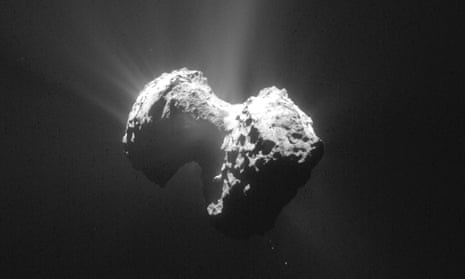This black and white image features a bright, rough-textured object at its center, set against a solid black background. The object, which resembles a porous space rock or asteroid, is characterized by numerous pits, cracks, and crevices. It appears to emit faint rays of light, with the most noticeable illumination coming from the top left. The light creates a contrast with the dark surrounding area, highlighting the rugged surface of the object. The rectangular image, predominantly dark, frames this centerpiece, which could be interpreted as a celestial body captured in a detailed, high-contrast photograph.